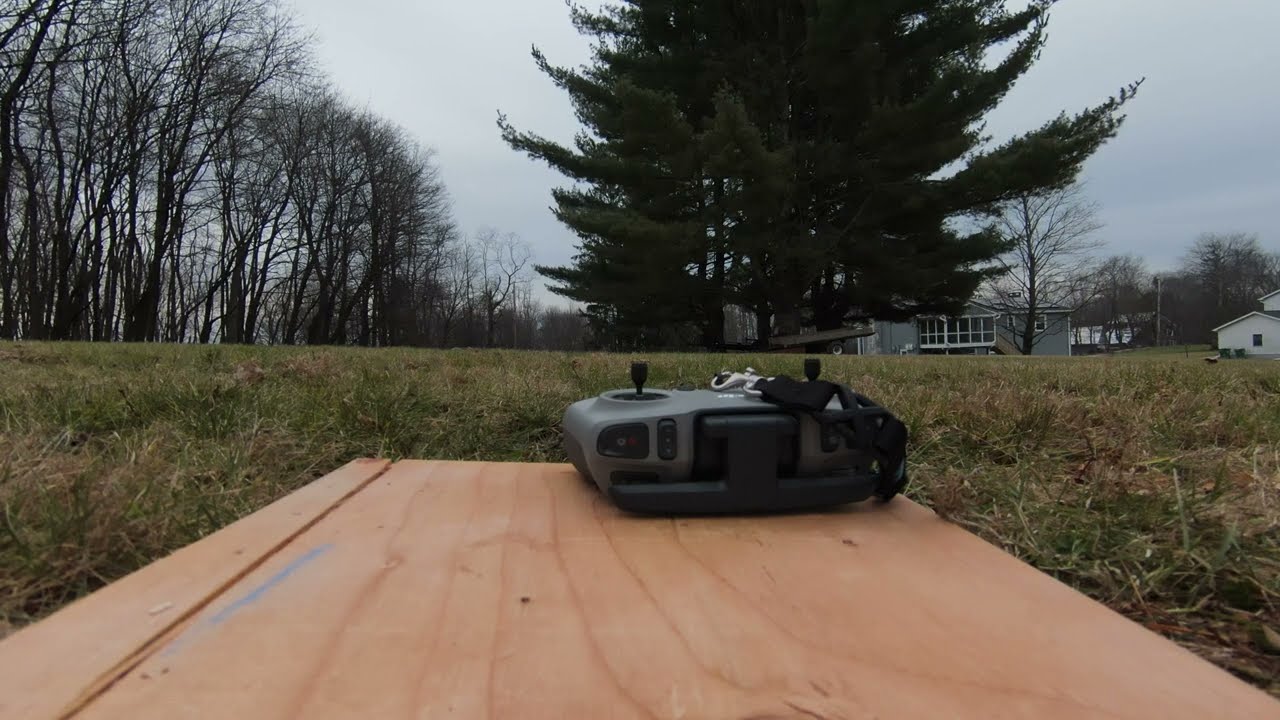This photograph captures a close-up outdoor scene taken from ground level, focusing on a mixed patch of grass that is primarily green with some brown due to dryness. In the foreground, there is a brown, square wooden board resting on the ground, upon which a black and gray RC controller with joysticks is prominently placed. Surrounding this setup, the landscape extends to reveal a mix of green and dry trees, suggesting a seasonal transition, possibly fall. The background includes two residential buildings: a small blue house with a covered porch resembling an all-season room, and a partially visible tan house with a garage. Tall pine trees are present, along with other trees devoid of leaves. The sky above varies between descriptions, with some saying it is blue with clouds, while others describe it as overcast, indicating perhaps a partly cloudy or changing weather condition. Overall, it is a daytime scene with a peaceful, slightly rustic ambiance.